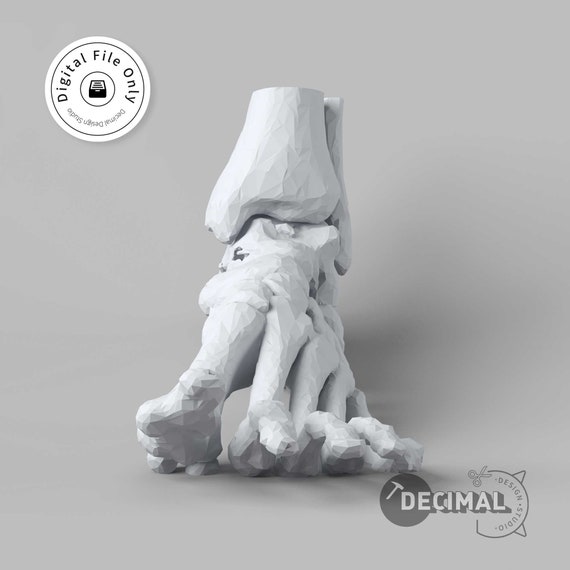The digital design features a detailed rendering of human foot bones, depicted in varying shades of white and gray on a gray background with subtle shadows. Prominently placed in the top left corner is a circle containing the text "digital file only." In the bottom right corner, there is a logo for Decimal Design Studio, highlighted by a gray rock hammer and scissors within a circular border. This highly detailed and monochromatic composition emphasizes the anatomical precision of the bones, showcasing each toe in a manner reminiscent of a white clay sculpture or possibly a plaster cast.